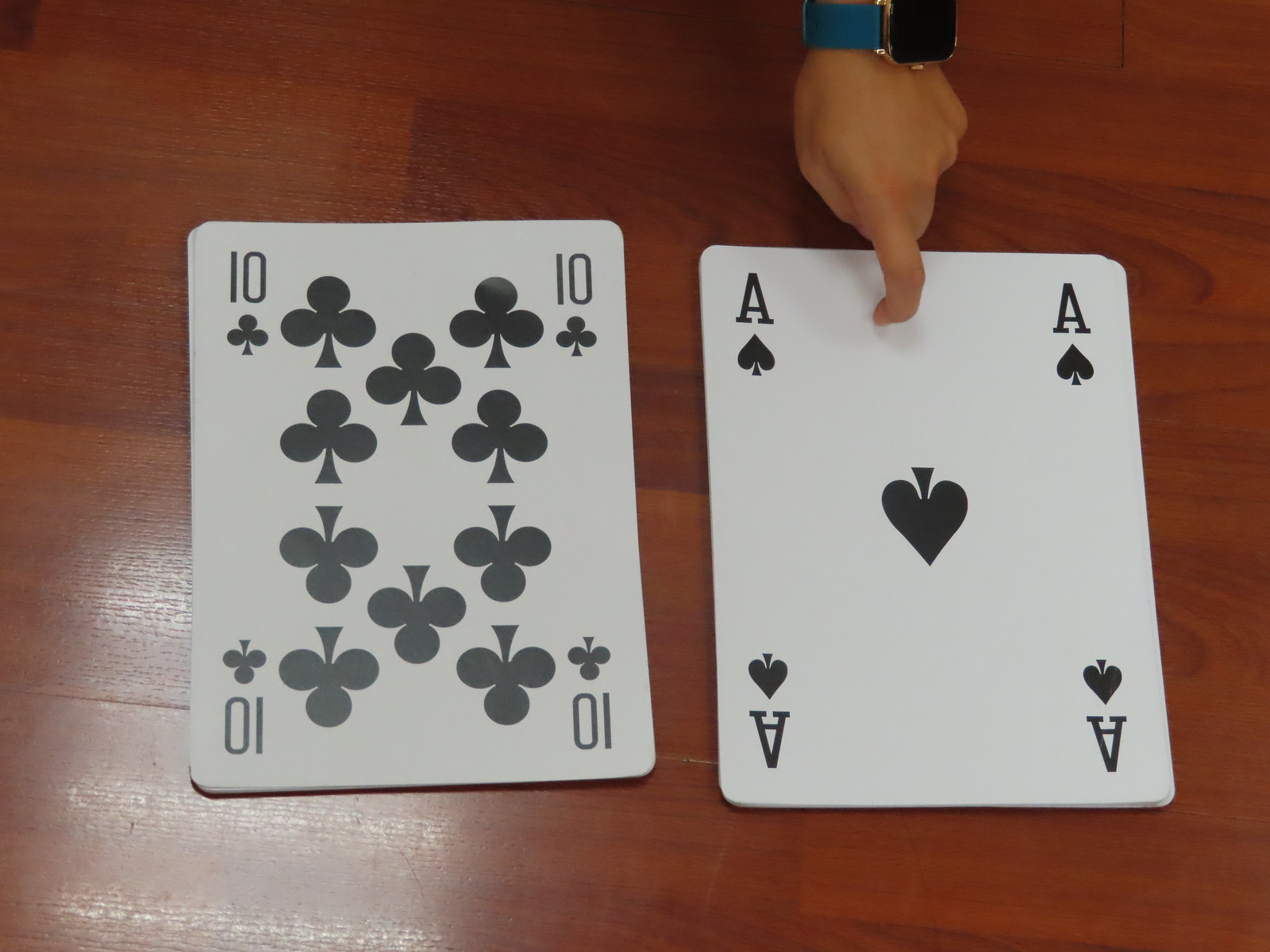This indoor photograph captures two towering stacks of oversized playing cards placed on a medium cherry wood floor. The left stack is topped with the ten of clubs, while the right stack displays the ace of spades prominently. The substantial size of the cards is evident from the presence of a Caucasian hand in the upper right corner, extending from the top of the frame. The hand, likely the left hand due to its positioning, is adorned with a wristwatch featuring a thick medium blue band and a square-faced silver smartwatch with a black face. The index finger of the hand is tapping the top of the ace of spades card, emphasizing the card's considerable dimensions; the hand appears almost half the width of the cards. Additionally, a light reflection is noticeable in the bottom left corner of the image, hinting at the overhead lighting.